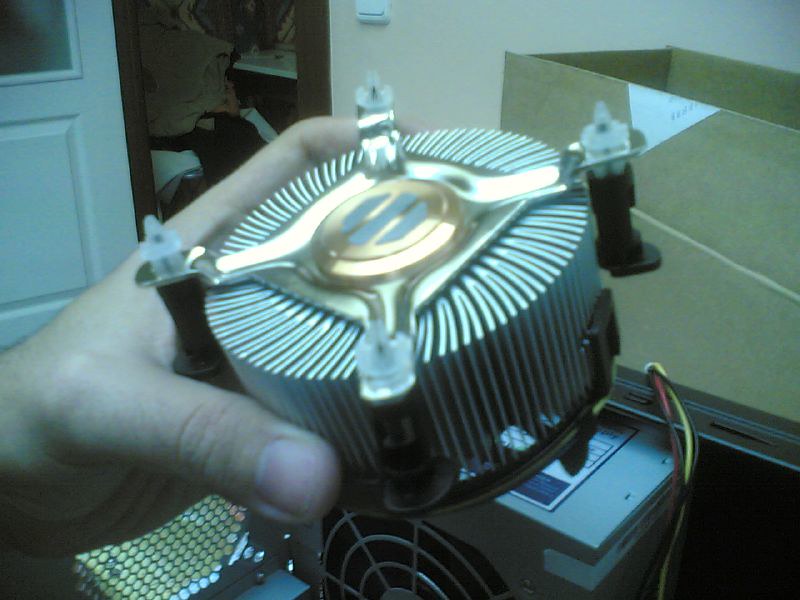In the image, a person's left hand, primarily using their thumb and pointer finger, is holding a circular component, likely a heatsink for a computer CPU. The heatsink is prominent in the picture, about twice the height of the person's thumb and approximately double the perimeter of the distance between their thumb and forefinger. The heatsink features a distinctive design, with tall V-shaped metal fins spiraling out from its center. Atop the heatsink, there's a gold square with a circular gold emblem in the middle, displaying three gray lines in a stylized pattern. Metal brackets radiate out from each corner of the gold square, where screws can be seen, suggesting it is designed to be mounted onto a PC case. The background appears to be a room or office space, indicated by a cardboard box and white walls. This setup, with its clear focus on the heatsink, suggests it might be part of a new PC build.